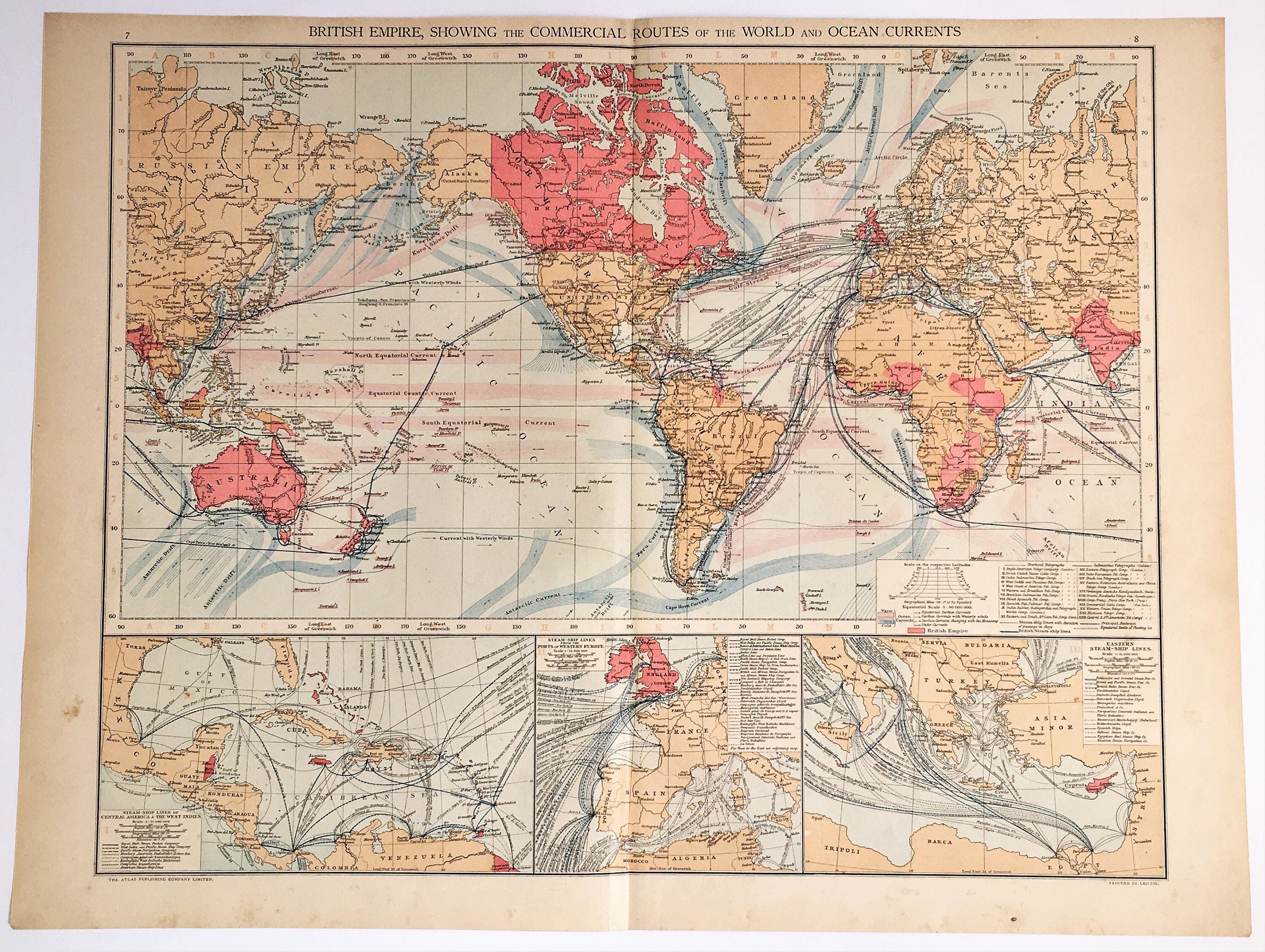This photograph captures an open book, displaying an old and weathered world map spread across two pages. The paper looks aged with a yellowed, tan hue and visible creases suggesting it has been frequently folded and unfolded. The top portion of the map prominently features a title: "British Empire showing the commercial routes of the world and ocean currents." 

The map highlights the British Empire territories in red, specifically Australia, Canada, parts of Africa, and India, while the rest of the world is depicted in orangey-tan, beige, and brown shades. There are also many blue lines illustrating ocean currents, some of which are a darker blue or light pink. Small, illegible black text details shipping lanes. 

In addition to the full world map, the bottom of the pages includes three smaller close-up images: one focuses on the Gulf of Mexico and the West Indies, highlighting areas like Mexico and Cuba; another zooms in on the shipping lanes between France and Spain, and the final inset looks at parts of the Mediterranean, including Asia Minor, Italy, and a portion of North Africa. 

Overall, this map provides an intricate view of global commercial routes and ocean currents as they were understood during the height of the British Empire, meticulously detailed on a worn and historical artifact.